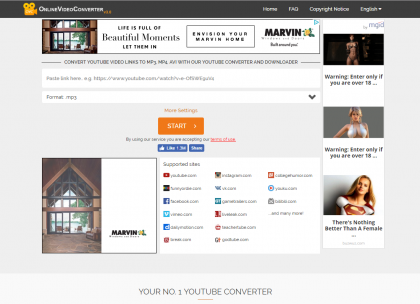This image is a small, somewhat blurry screenshot taken in landscape mode, containing several distinct sections. It has a dark stripe running horizontally across the top. On the upper left is a partially legible business logo that appears to resemble a movie camera. The upper right contains navigational options: "Home," "FAQ," "Copyright Notice," and "English."

Below this header, there's an advertisement with the slogan, "Life is full of beautiful moments – let them in," which appears to be promoting Marvin Windows. The next section offers a service to convert YouTube video links to MP3 or MP4 formats using a YouTube converter and downloader. This section is set against a gray-on-white background, making it challenging to read.

Following that, there are options for conversion format, with MP3 selected and a dropdown menu available. To the right, an orange "More Settings" button is visible, accompanied by a prominent orange "Start" button. Below this, a red link and blue buttons for Facebook Like and Share are present.

On the right-hand side of the image are advertisements that seem to lead to adult content. They carry warnings such as "Enter only if you are over 18" and messages like "There's nothing better than a female," indicating potentially sexist and pornographic nature.

At the bottom of the image, the site brands itself as "Your Number One YouTube Converter."